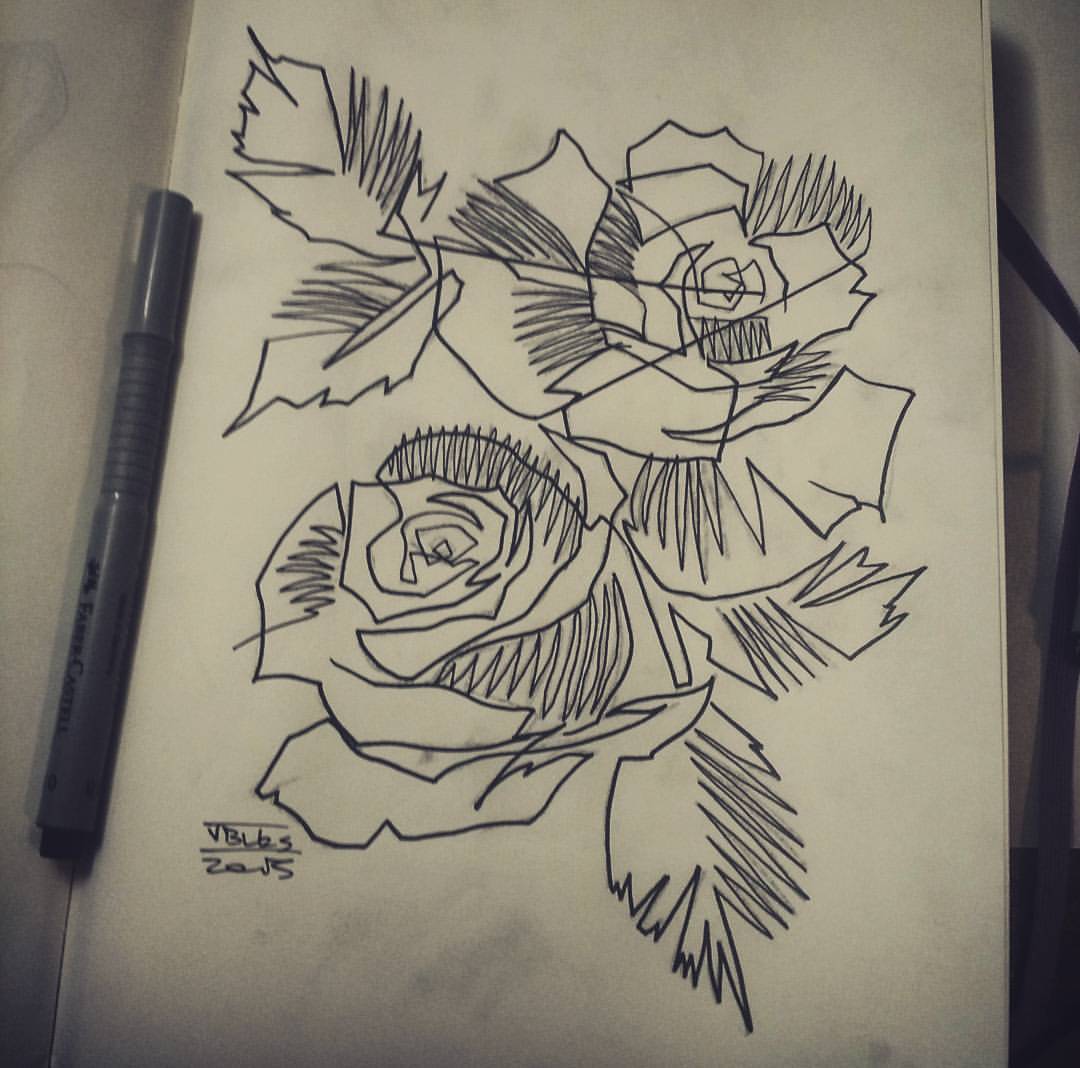This photograph captures a detailed pen sketch of stylized roses in an off-white notebook. The drawing features two abstract-styled roses, each with intricate, zigzagging petals and sharply serrated leaves. The roses are positioned with one leaning towards the top right and the other slightly lower, facing the top left. Each rose is accompanied by two leaves, one pair in the bottom right and the other in the top left. The artist has added shading using long zigzag lines, creating a textured effect. There is a noticeable smudge on the image, and a gray pen, likely used for the drawing, is placed in the crease of the open notebook, its lid on. This sketch, signed with what appears to be "VBLBS ZERS" or "2015 in B Books," is captured in a somewhat blurry, black and white photograph that shows the elastic band of the sketchbook on the right edge.